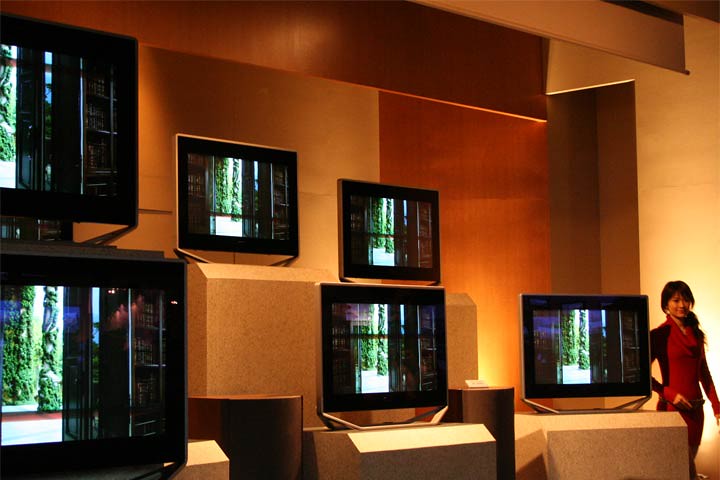The photograph features an ambient, dimly lit room with a brown wall in the background that gives a 3D visual effect with its dimensional shapes. The central feature is six futuristic, flat-screen television monitors, organized in two rows of three, each on modern, stone-slab-like stands. All screens display the same image of a window overlooking a lush, green, tree-lined area. In the bottom right corner, an Asian woman, possibly in her 20s, with long brown hair wearing a long-sleeved red dress or shirt, stands facing the camera. The setting appears to be a store or showroom, with dramatic lighting enhancing the overall warm and sophisticated atmosphere.